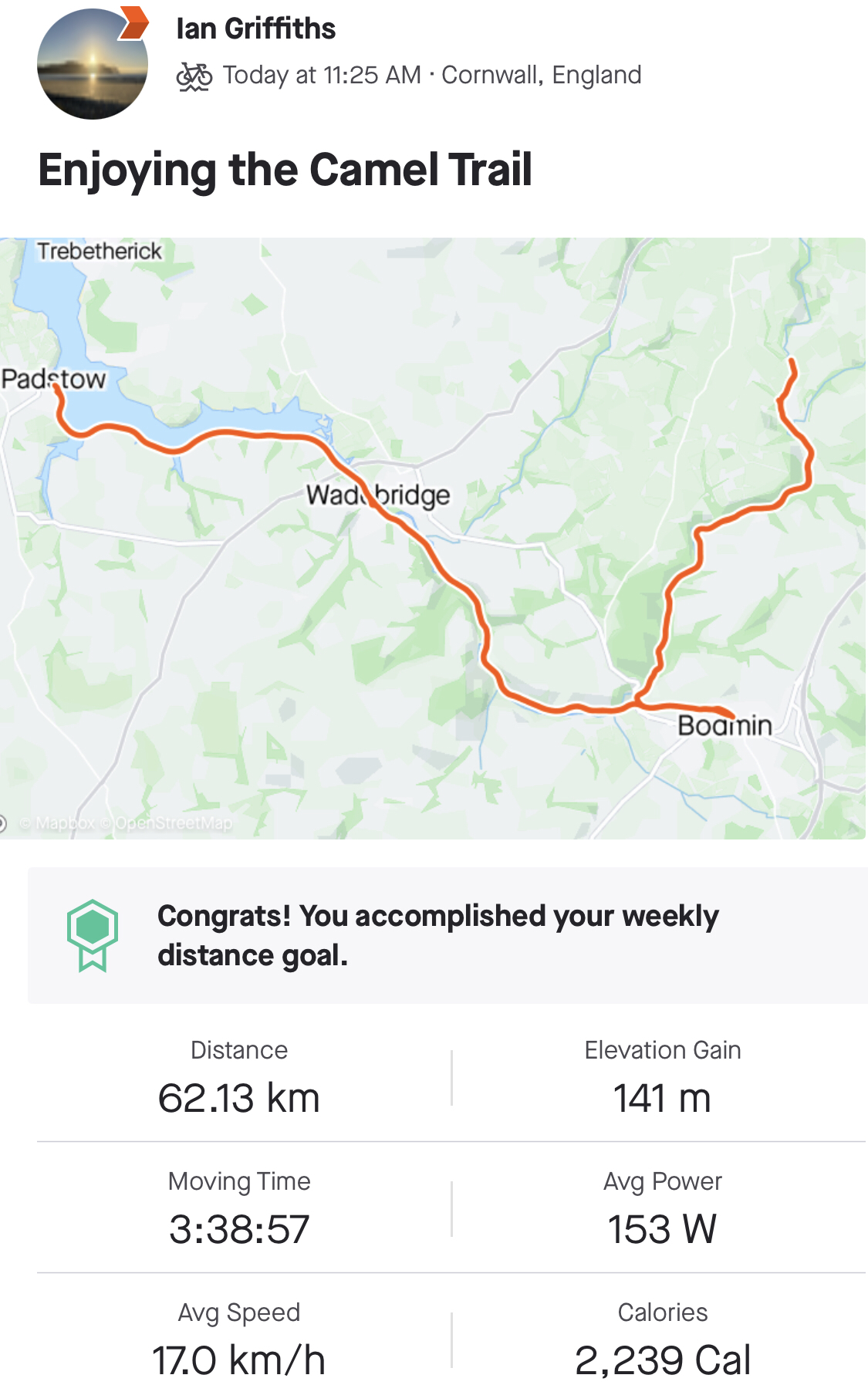The image is a horizontally oriented snapshot of an app interface displaying cycling statistics and a route map. At the top eighth of the image, there's a white banner reading "Ian Griffiths" in bold black font, positioned about an inch from the left. Below Ian's name, a small black bicycle icon is visible, along with finer text that states, "Today at 11.25am - Cornwall, England."

Adjacent to this text, on the left, there’s an oval image of a sunrise, with a red arrow pointing to the top-right corner of the oval. Underneath, in large black text, it reads, "Enjoy the Camel Trail." 

The map below this header is depicted in shades of greyish-blue with green accents, featuring a highlighted red trail that winds along a river. Key locations marked in small black font include "Trebetherick" at the top right, "Polzeath" near the river's wider section, "Padstow," "Wadebridge" at the midpoint, and "Bodmin" towards the map's bottom.

Beneath the map, a light blue banner features a green award icon on the left, followed by the congratulatory message, "Congrats, you accomplished your weekly distance goal" in mostly lowercase letters. Detailed performance metrics are displayed in two columns beneath the banner:

- **Distance:** 62.13 km
- **Moving Time:** 3 hours, 38 minutes, and 57 seconds
- **Average Speed:** 17.0 km/h
- **Elevation Gain:** 141 meters
- **Average Power:** 153 W
- **Calories Burned:** 2,239

The app interface combines meaningful text and visual elements to provide a detailed record of a cycling session on the Camel Trail in Cornwall, England.